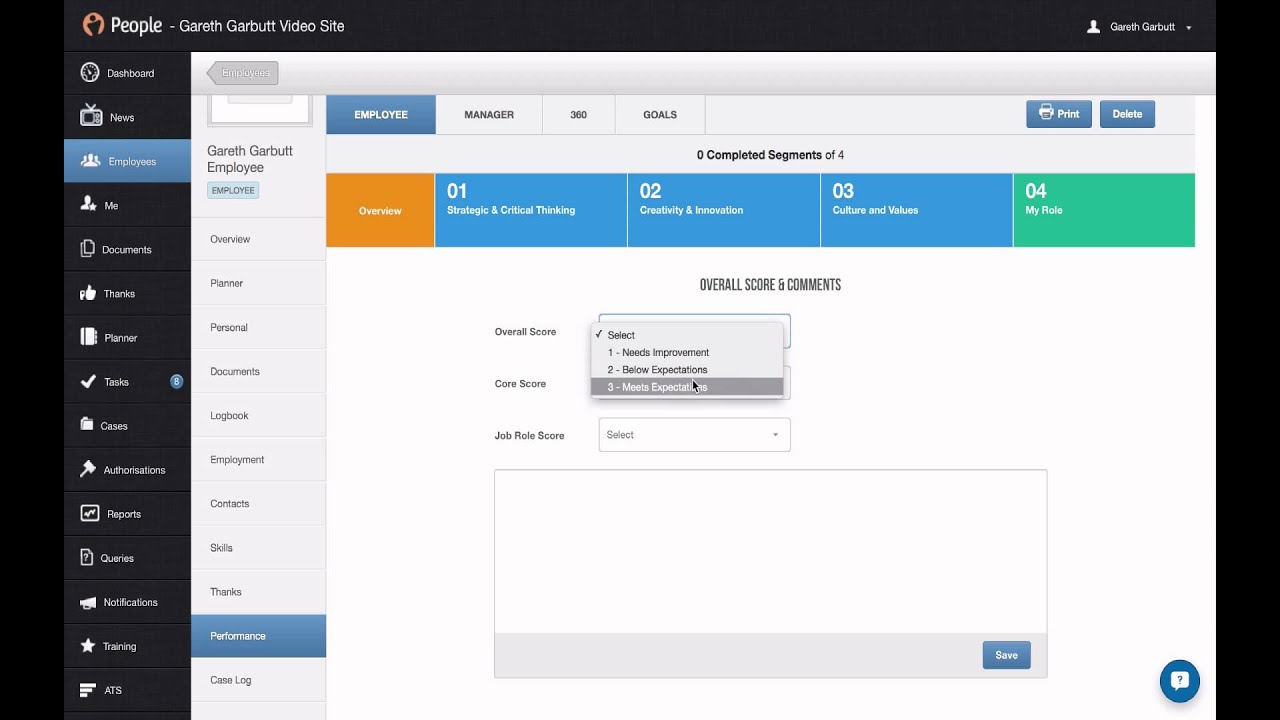The image is a detailed screenshot of a webpage from Gareth Garbutt's video site, as indicated by the page header. Along the left-hand side, there's a vertical menu with various options including Dashboard, News, Employees, Me, Documents, Thanks, Planner, Tasks, Cases, Authorizations, Reports, Queries, Notifications, Training, and ATS.

In the main part of the screen, enclosed within a black box, is a highlighted section with the label "Gareth Garbutt Employee." This section includes tabs for Employee, Manager, 360, and Goals, allowing users to navigate through different view options.

On the right side, there are small blue buttons labeled Print and Delete. The central part of the page seems to function as an evaluation tool. It starts with an Overview tab in an orange box, followed by evaluation categories: 01. Strategic and Critical Thinking, 02. Creativity and Innovation, 03. Culture and Values, and 04. My Role (green box).

In the middle of the evaluation section, it includes fields for Overall Score and Comments. Each score field is accompanied by a drop-down menu with options such as Select, Needs Improvement, Below Expectations, and Meets Expectations. There are additional dropdown fields for Core Score and Job Score.

A text area is provided for written notes, and there is a save button at the bottom to save the entered information.